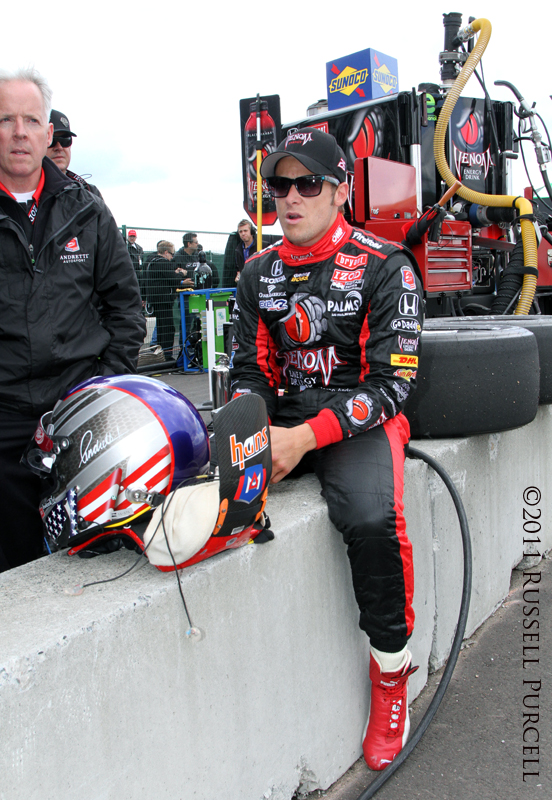The image captures a detailed scene at a racing event in the middle of the day. Centered in the photo, a race car driver is seated on a stone or cement wall, with his legs dangling over the edge. He sports a dark racing suit adorned with various advertisements and features red trims, complemented by dark pants with a red sash and red shoes. A large helmet with silver, blue, and red accents sits just in front of him on the wall.

In the background, a packed crowd of spectators can be seen, some seated in bleachers, indicating the race's popularity. Various objects around them include tires and items commonly used in pit stops, along with a stand or scoreboard and a Sodonko sign. The backdrop provides a vibrant outdoor setting typical of a race track, with scattered colors of light gray, dark gray, black, red, yellow, orange, blue, and green. A copyright mark at the bottom reads "2011 Russell Purcell." Overall, the image vividly captures the bustling atmosphere of a race day, highlighting the driver's moment of pause amidst the high-energy environment.